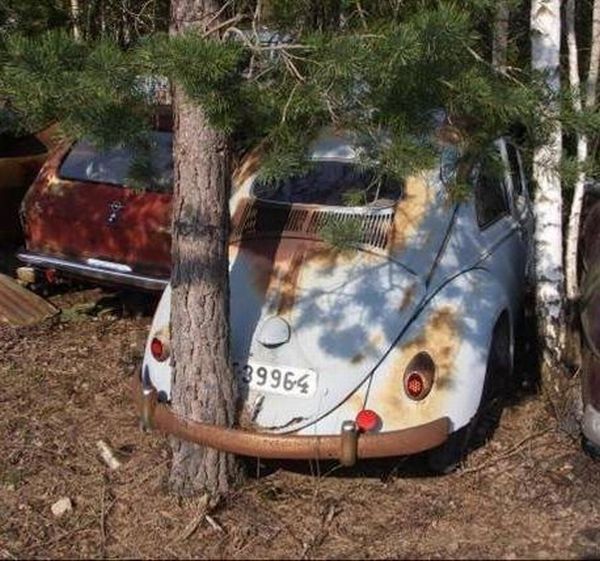The image depicts a haunting scene of two old, abandoned vehicles amidst a dense, wooded area. At the center-right, there is an aged, light-colored car, likely a rusted Volkswagen Beetle, with its corroded rear bumper embracing a tree trunk, which is adorned with sparse green pine needles. This peculiar entanglement suggests the car has been forsaken for quite some time. To the left of this scene is another forgotten vehicle, a dark red hatchback, also showing signs of significant aging and disuse. The ground beneath them is a brown carpet of dirt, scattered with loose sticks and branches, contributing to the desolate atmosphere. Surrounding the cars are various trees, including thin, white birch trunks to the right, and more foliage in the background, immersing the entire scene in a natural, yet eerie, woodland setting. The diagonal positioning of the cars adds depth to the composition, emphasizing the passage of time in this somber tableau.